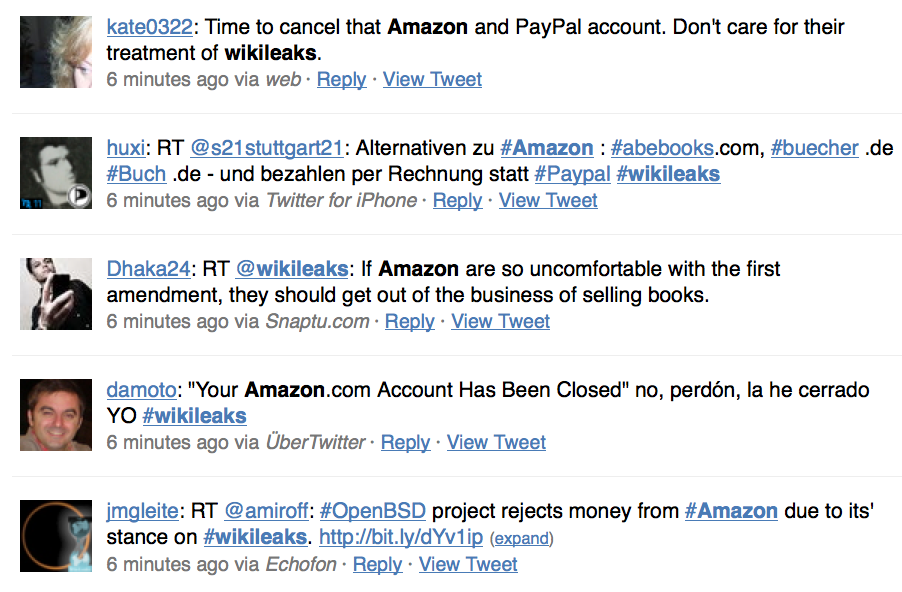The image appears to be a screenshot of a Twitter comment section featuring user names and their tweets, all displayed in a vertical column. On the left side of the image, there is a white background with five small profile photos, each corresponding to a different user. The first user, "Kate0322," with blonde hair and half of her face visible, has posted a tweet six minutes ago saying, "Time to cancel the Amazon and PayPal account. Don't care for their treatment of WikiLeaks." Both her username and the "reply" and "view tweet" links are displayed in underlined blue text. The second user, "Huxy," who has black hair and a black background, has posted a tweet in another language also from six minutes ago. Following that is a user named "DACA24" holding a cell phone, with a tweet mentioning retweeting alternatives to Amazon due to their stance on WikiLeaks. Beside the fourth photo, "D'Amato" has posted in Spanish about closing an Amazon account. The last user, "J-M-G-L-E-I-T-E," has a tweet that criticizes Amazon for its treatment of WikiLeaks and suggests that if they are uncomfortable with the First Amendment, they should not be in the business of selling books. Each entry includes the underlined blue text for "reply" and "view tweet," reinforcing the Twitter format.